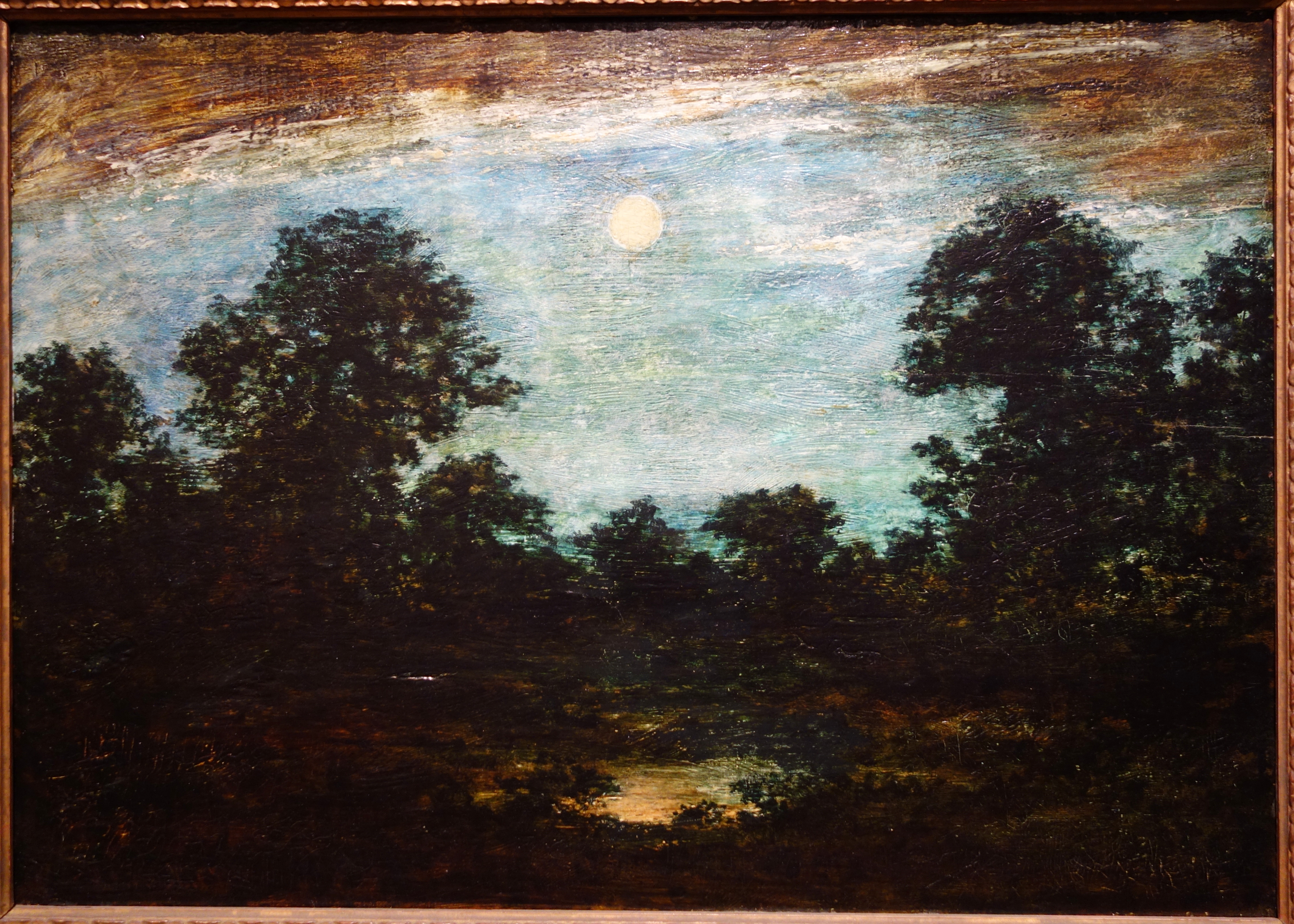This dark oil painting depicts a nocturnal scene illuminated by the moon. The composition is dominated by nearly black trees with dark greenish hues, encircling a small, light brown clearing that might suggest a grove. The upper central part of the painting features a white circle, presumably the moon, casting its glow upon the landscape below. The sky transitions from a medium blue, tinged with the subtle light of the moon, to darker brown tones higher up, with gray smudges adding to the night-time ambiance. Below the sky, a minuscule lake or pond, surrounded by shrubbery and tall trees, reflects the moonlight, giving the water a brownish tint except where it mirrors the lunar glow. The painting appears to be an image of an oil painting, as part of the ornate brown frame is visible around the edges. The primary focus is the moonlit grove and its ethereal illumination against the dark, wooded surroundings.